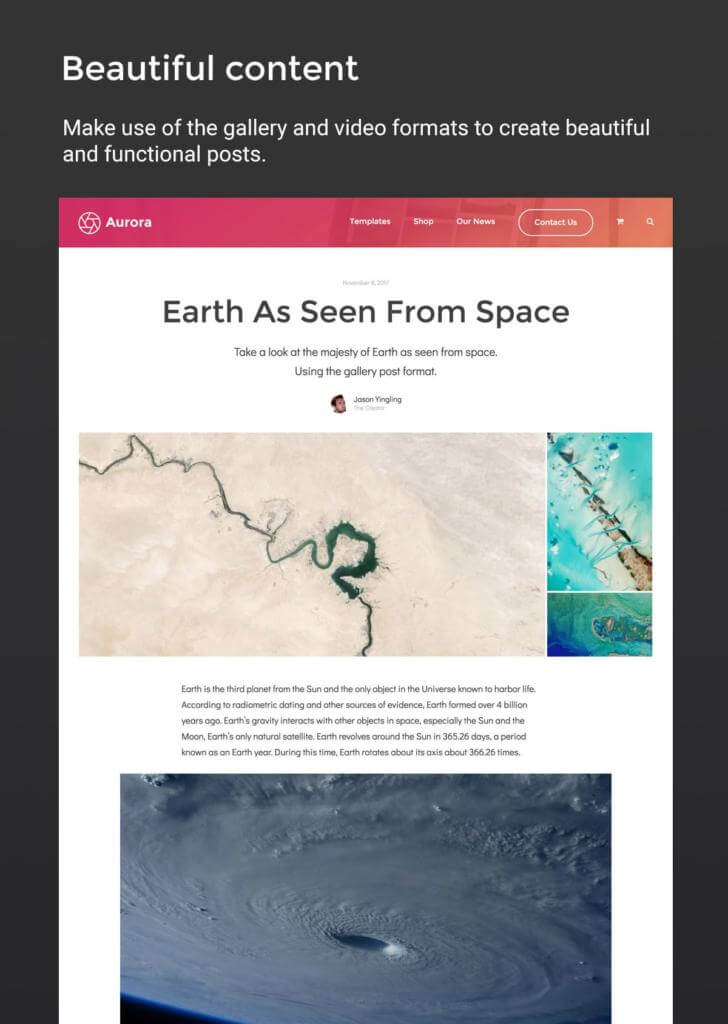The image portrays a presentation with a sleek, black background, topped with the phrase "Beautiful Content" in bold, white text. Below this header, there's a guiding suggestion: "Make use of the gallery in video formats to create beautiful and functional posts."

The focal point is a prominent red rectangle, inside which the word "Aurora" is boldly typed. Directly beneath this, in crisp black text, reads the subtitle "Earth as seen from space," setting the context for the captivating visuals below.

The image further features a striking visual—a vast expanse of a white mass, traversed by a green line that gradually thickens toward the base, reminiscent of a crack in a snowy landscape. To the right of this, an intricate image showcases vibrant blue water intersected by a distinct brown line down its center, juxtaposed with another perspective of the ocean below. This portion of the image transitions from a deep, dark blue hue on the bottom left to a more vibrant turquoise on the right.

Accompanying these visuals is a concise informational paragraph in very small black text.

Lastly, the composition includes a view from space, displaying a swirling mass of white smoke with a distinct dark blue section in the bottom left corner, encircling a central area, evoking the ethereal beauty of our planet seen from the cosmos.